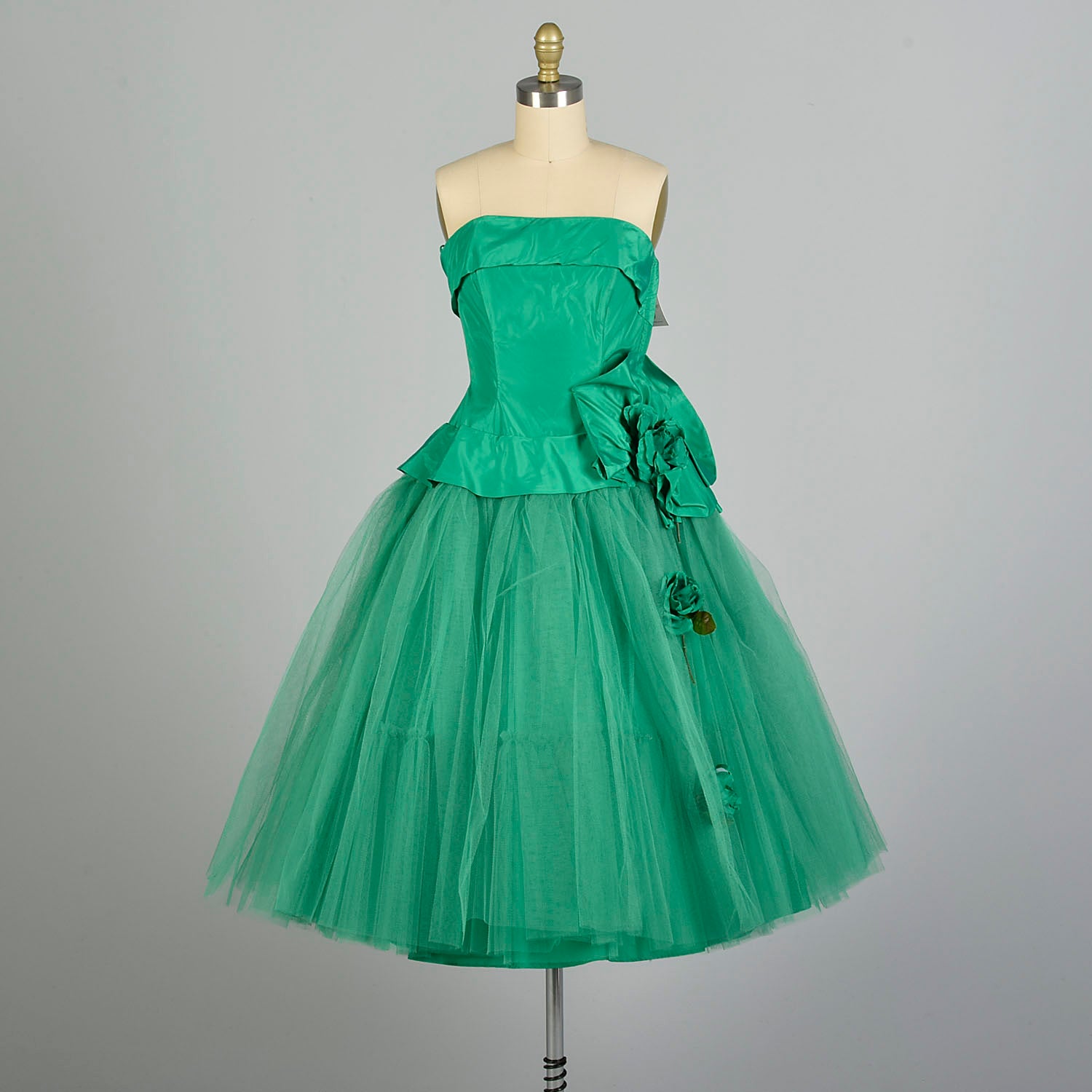This color photograph features a sleeveless dress displayed on an ivory dressmaker's model that has no arms or head but is topped with a gold accented knob. The mannequin is held up by a silver rod and stands against a solid gray background, where the gray shifts from lighter shades in the center to darker tones in the corners.

The dress itself is a striking teal, described variably as turquoise and dark lime green. It consists of a shiny, solid fabric around the bust, and transitions into a multi-layered, heavily folded skirt made of thin, sheer fabric reminiscent of a long tutu. A distinctive element of the dress is a loose, abstract piece of solid fabric from the bust portion, pinned to the waist on the right side, possibly intended as a large bow or a stylistic flower. Another similar decorative feature, described as material green roses or flowers, adorns the left side of the waist, adding an artistic touch to the garment.